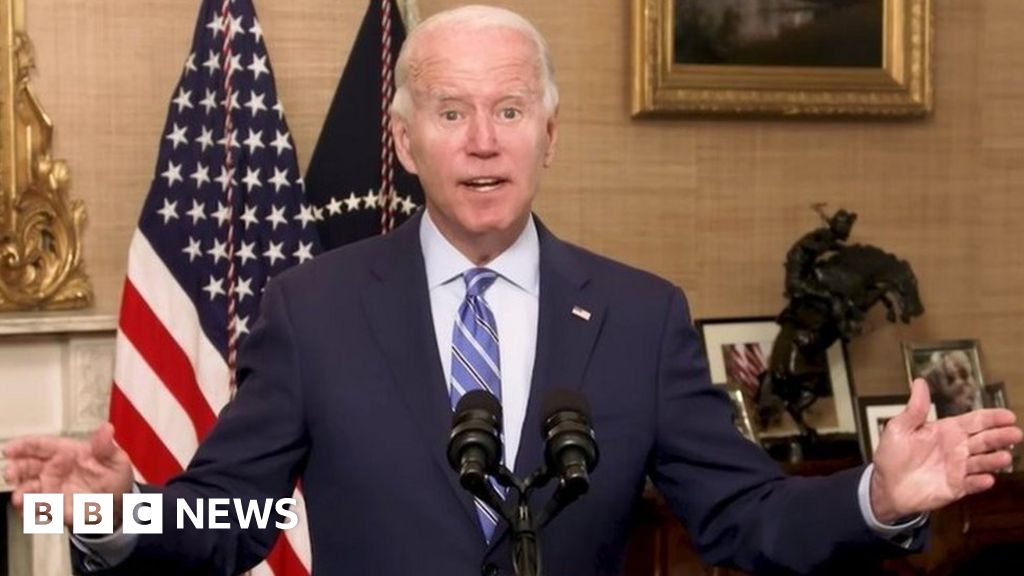In this detailed image, President Joe Biden is seen delivering a speech. He is dressed in a navy blue suit, paired with a white collared shirt, and a blue tie adorned with black and white stripes. The President stands with his arms outstretched in a gesturing manner, his mouth open as he speaks, and a concerned expression with wide eyes. In front of him, there is a double microphone setup. The backdrop includes two American flags and a light brown textured wallpaper with a white mantle featuring a gold decorative border. To the right, a tabletop holds a bronze statue of a man on a rearing horse and several framed photographs. Above this setup, a gold-framed piece of artwork is visible. The bottom left corner of the image bears a white "BBC News" logo, indicating this is a screenshot from a newscast.